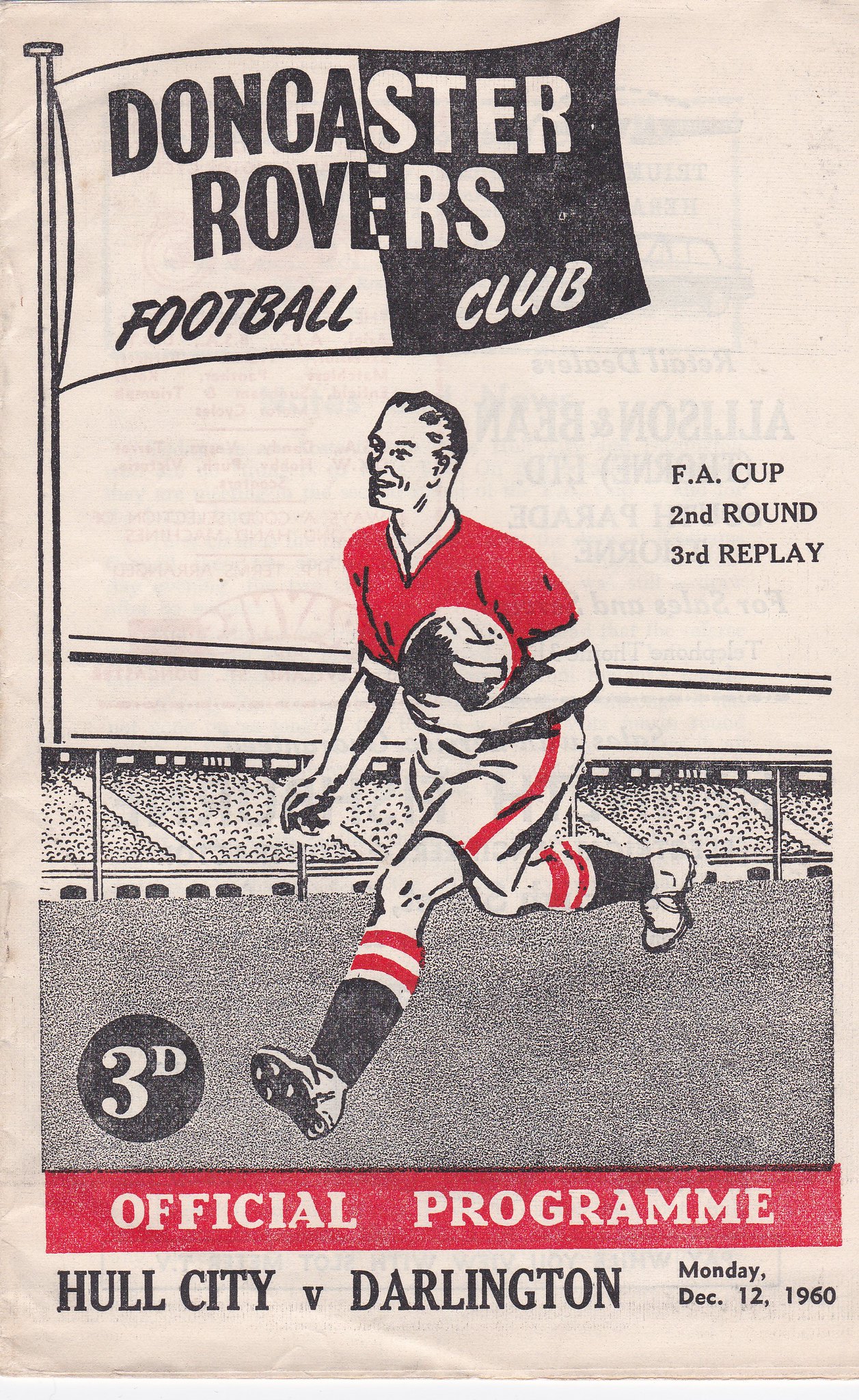This is a vertically aligned rectangular cover of an official program for the Doncaster Rovers Football Club, featuring multi-color print on off-white stock. The left side of the cover, acting as the spine, displays a large flag divided into black and white segments. The flag prominently features the text "Doncaster Rovers Football Club," with the words split so that "Donca" and "Football" are on the white background and "Rovers" and "Club" are on the black background. In the center of the cover is an illustrated soccer player dressed in a red shirt with white shorts accented by a red stripe, running with a soccer ball on a field towards the viewer. The player is accompanied by a huge black and white flag overhead. On the right, black text reads: "FA Cup Second Round Third Replay." Near the bottom left sits a black circle with the white text "3D" inside it. Below this, a red rectangular section houses the white uppercase text: "Official Program." Directly beneath this, in black text, it reads: "Hull City vs. Darlington," with the date "Monday, December 12, 1960," positioned at the bottom right. The entire scene is depicted as a drawing, giving it a distinct illustrative style.